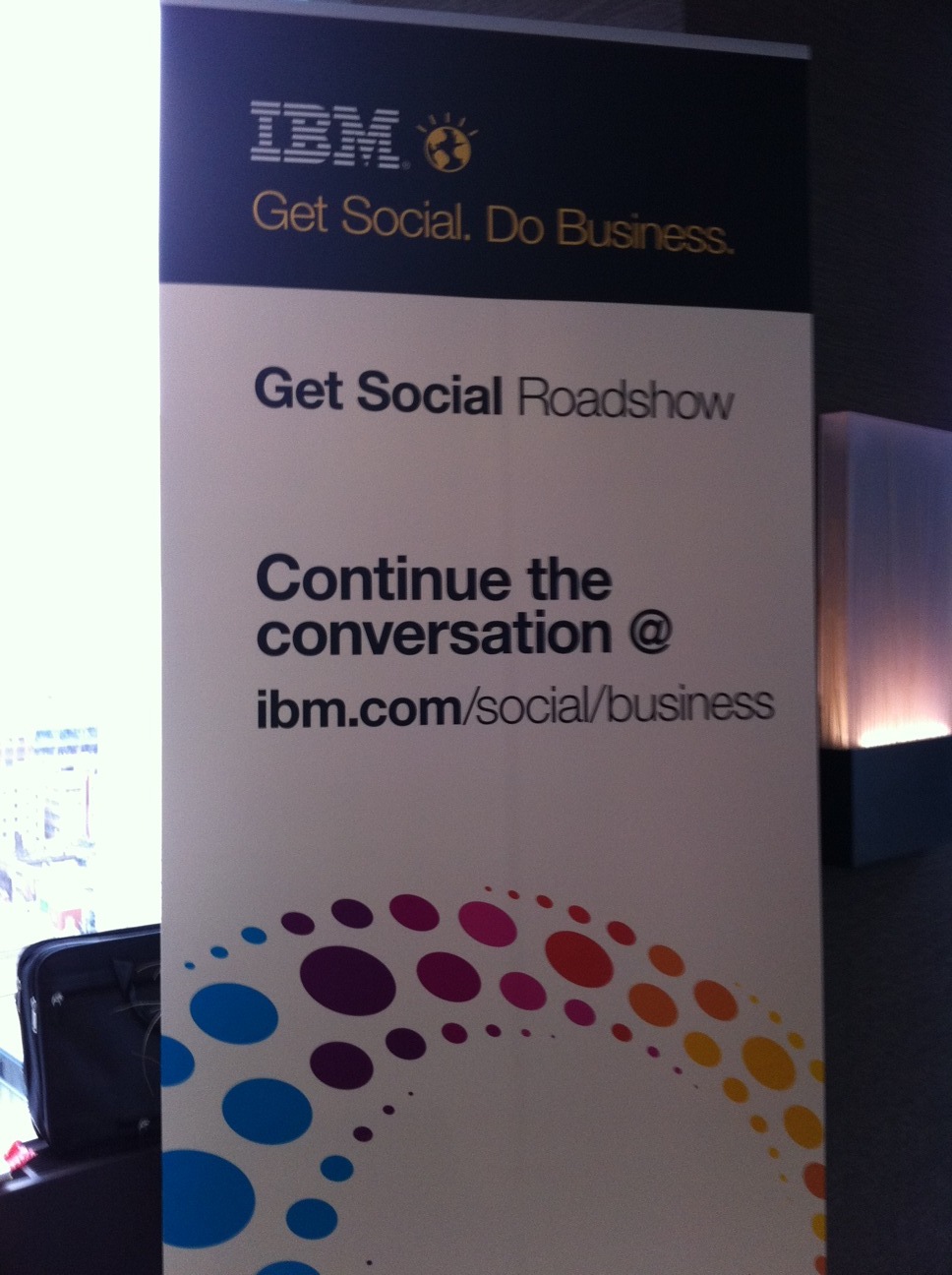This large, eye-catching poster prominently features IBM's "Get Social. Do Business." campaign. The title, in bold blue text, is at the top of the poster. Centrally displayed is the phrase "Get Social Roadshow," indicating the event being promoted. Below this, the poster invites viewers to "Continue the conversation at ibm.com/social/business." The layout of the poster is predominantly white, but the lower half boasts a vibrant, polka-dotted rainbow design featuring blue, purple, pink, orange, and red dots. This colorful section likely aims to attract attention and emphasize the dynamic nature of the event. The overall appearance suggests that the poster is intended for display at a store or conference to promote IBM's social business initiatives and their ongoing roadshow.